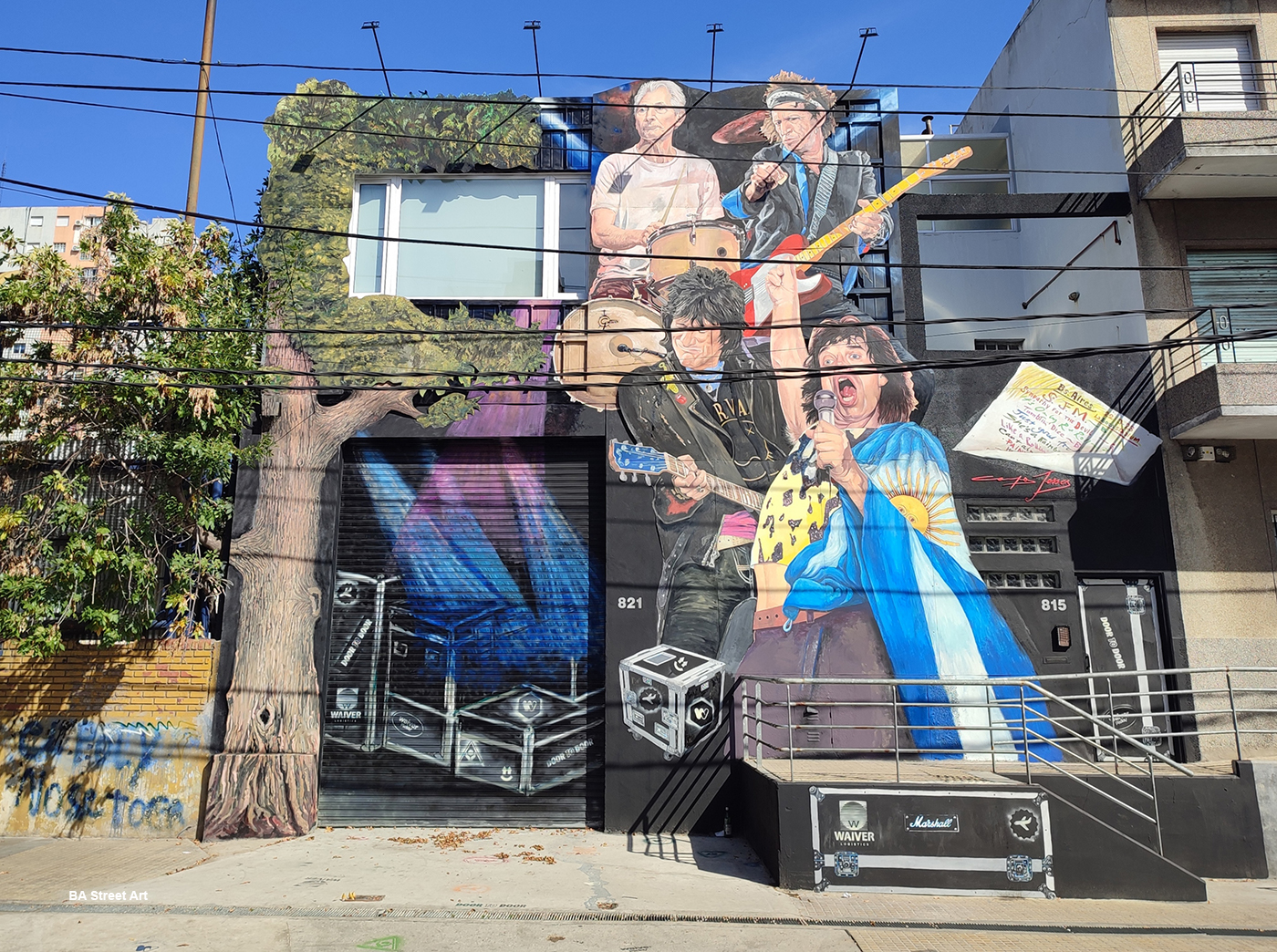This image captures a vibrant daytime scene of a building adorned with artistic murals. The structure, which appears to be an apartment or condo building, features a stone facade with terraces and multiple dwellings. Prominently displayed on the exterior is an expansive mural dedicated to the Rolling Stones, showcasing detailed portraits of Mick Jagger singing into a microphone, along with the band's guitarist, bassist, and drummer, all in various poses that convey energy and movement. The mural also includes painted speaker boxes and musical equipment, amplifying the rock 'n' roll theme.

The entire building is painted over in black, with additional artistic elements such as a tree whose trunk and branches curve up the left side, framing a window. The numbers 821 and 815 are visible, indicating different units within the building. At the lower left corner of the image, the text "Be A Street Art" is visible, adding to the artistic vibe. This lively mural transforms the building's facade into a dynamic homage to music and art, making it stand out in its urban environment.